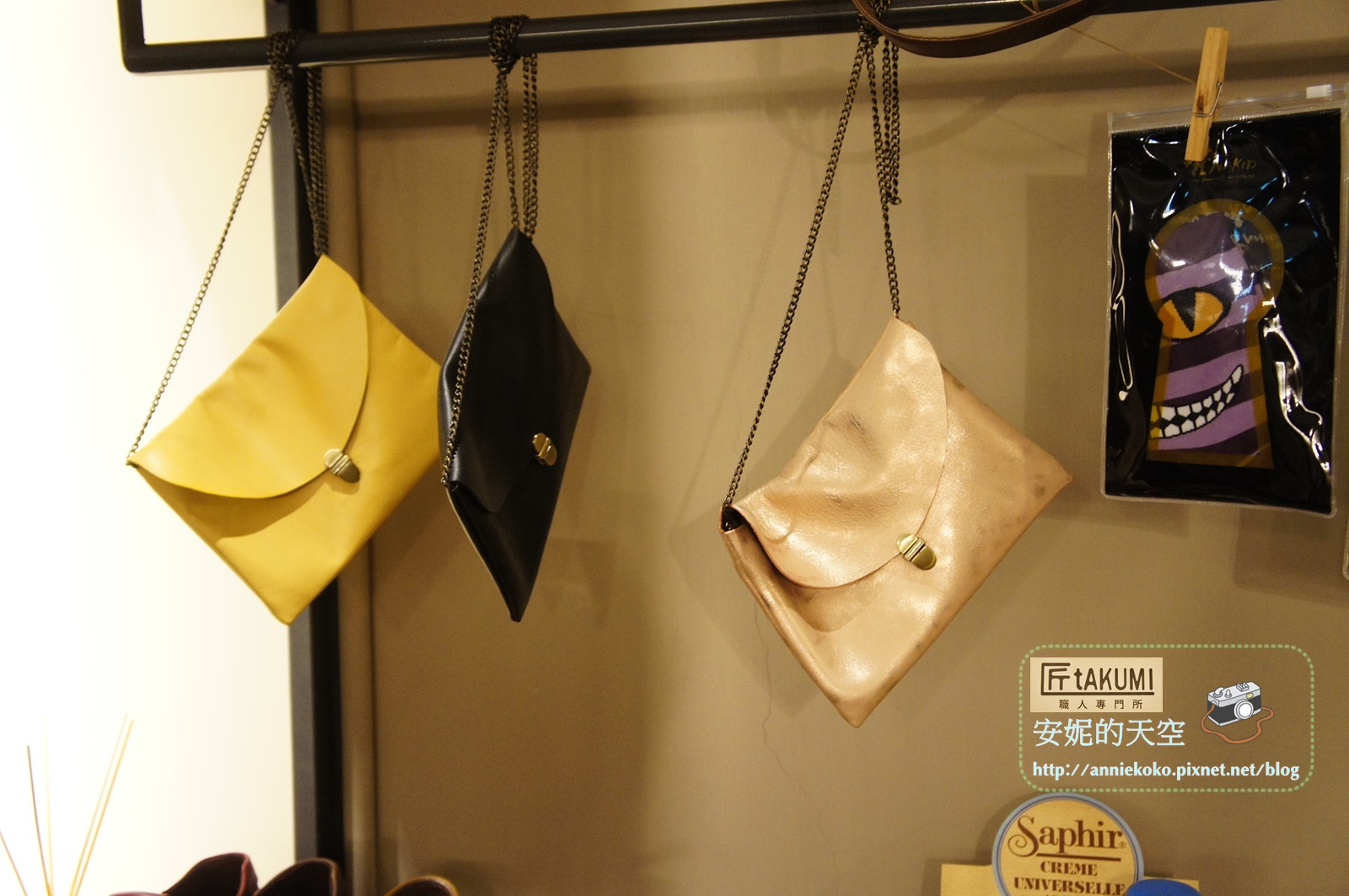The image depicts a store display featuring three leather purses hanging on chains from a horizontal black pole. The purses, which come in yellow, black, and tan, are arranged in a way that showcases their different styles—two having front clasps, and one appearing to zip along the top. Below these purses, there is a small display featuring a container labeled "Saphir Crème Universelle." Additionally, a peculiar piece of art, resembling a cartoon face, dangles by a wire clipped with a clothespin from the same pole. The background wall is beige, and a black purse with a print resembling a Cheshire cat hangs in the corner, also attached with a clothespin. At the bottom right corner of the photograph, there is a watermark or logo that reads "Anikoko.pixnet.net/blog" along with some Japanese kanji characters. A black plastic bag is visible on the right side of the image, though its contents are unclear.